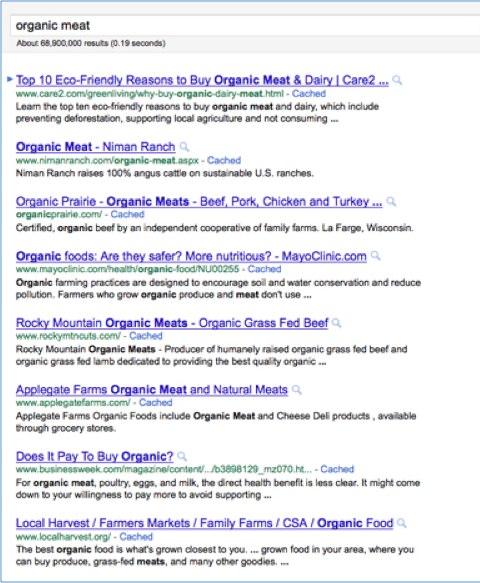In this cropped image of a search engine, possibly Google or Yahoo, the focus is on search results for the query "organic meat." The search yielded approximately 68 million results in about 0.19 seconds. The results displayed include a mix of informational articles and potentially advertisements. The search results feature titles such as "Top 10 Eco-Friendly Reasons to Buy Organic Meat and Dairy," "Organic Meat," "Organic Prairie Organic Meats," "Organic Foods: Are They Safer, More Nutritious?" by Mayo Clinic, "Rocky Mountain Organic Meats," "Applegate Farms Organic Meat and Natural Meats," "Does it Pay to Buy Organic?" by Businessweek.com, and "Local Harvest Farmers Markets Organic Food" by localharvest.org. Each search result listing includes the full website URL below the title, followed by a "Cached" link, and beneath them, a brief description of the website's content.